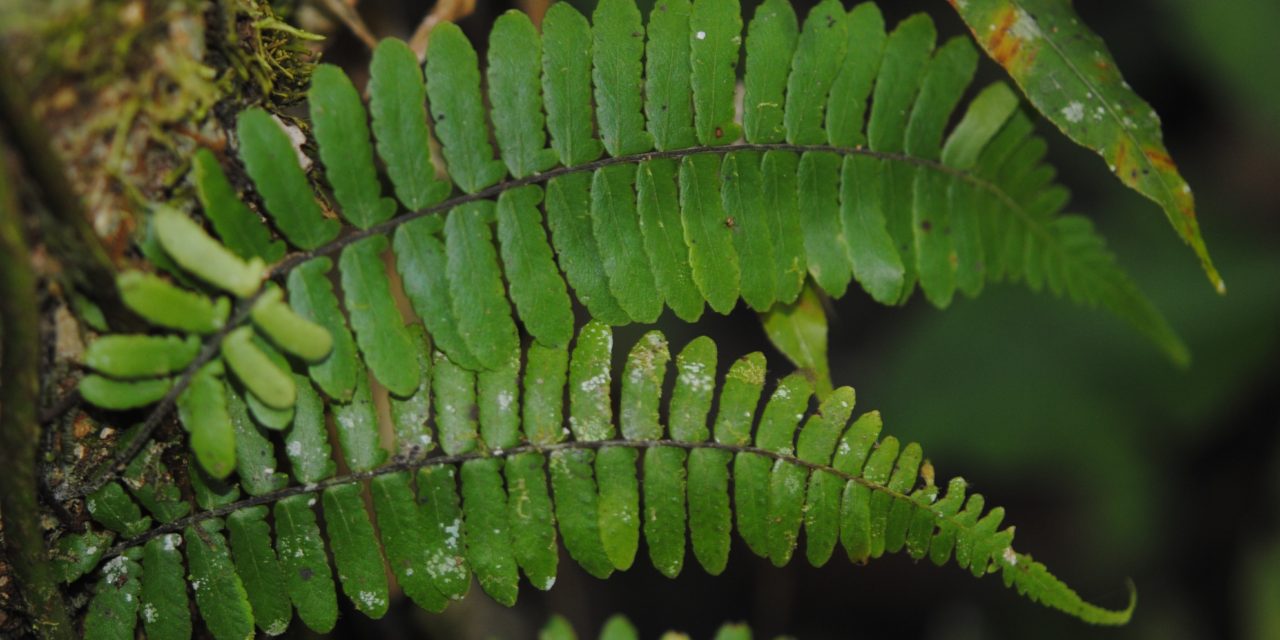This close-up image captures several fern leaves stretching diagonally across the frame. The leaves, mainly a vibrant dark green with occasional flecks of dirt, emerge from a patch of soil and dirt situated on the left-hand side. The topmost fern leaf appears the healthiest, showcasing a vivid green color, while the bottom fern leaf exhibits some white markings, potentially indicating damage or disease. In the image, the fern's characteristic structure is clear, with individual fronds each shaped like a peanut, connected to a central stalk. Among these fern leaves, towards the upper right, there is also a more traditional leaf with visible veins and slight brown and yellow discoloration. The background on the right-hand side of the photo is notably blurry, enhancing the focus on the fern leaves and hinting at an outdoor setting with natural light. The exact origin of the ferns—whether from the ground, a bush, or a tree—remains ambiguous due to the angle of the shot.